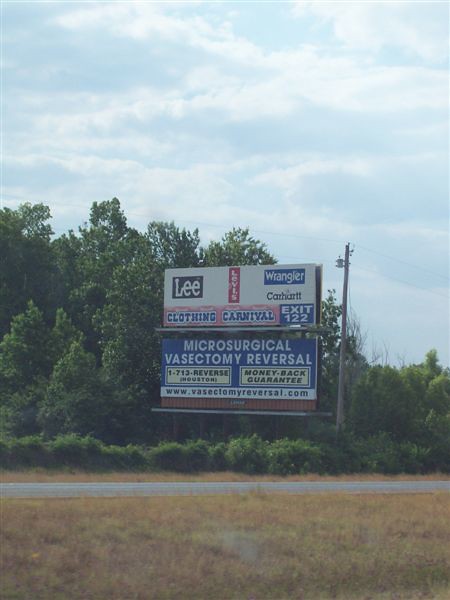In this photograph, the primary focus is on two juxtaposing billboards under a clear, light blue sky adorned with fluffy white clouds. The background features a scattering of deciduous trees, hinting at a rural or suburban setting. Below the billboards lies a blacktop road bordered by patches of browned grass, suggesting either drought or seasonal change. The overall image appears slightly washed out, possibly due to the age of the photograph or the intensity of sunlight.

The top billboard prominently advertises a "Clothing Carnival" located at Exit 122, with brand names like Lee, Levi's, and Wrangler vividly displayed. Meanwhile, the lower billboard presents a stark contrast with its advertisement for a "Microsurgical Vasectomy Reversal." It lists a contact number, "1-713-REVERSE," and boasts a money-back guarantee, providing a web link, www.vasectomyreversal.com, for further information. A faint line delineates the lower section of this billboard, revealing brown and gray hues. To the right of the billboards, a solitary telephone pole stands with faintly visible wires extending across the scene, adding an element of connectivity to the otherwise static tableau.